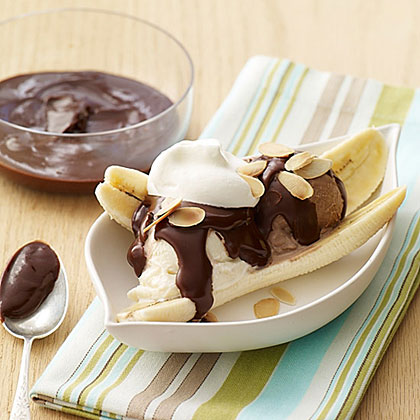This color photograph features a delectable banana sundae in a leaf-shaped white serving dish. The banana, sliced lengthwise into quarters, serves as the base for generous scoops of vanilla and chocolate ice cream. The ice cream is drizzled with rich, brown chocolate fudge and garnished with sliced nuts, which could be slivered almonds or possibly cashew shavings. At the center, a small dollop of whipped cream crowns the dessert. The sundae is elegantly placed on a folded kitchen towel that displays a blue, green, brown, and white pattern. In the back left of the scene, there's a small bowl containing extra chocolate fudge. Additionally, a silver spoon with a dollop of fudge rests in the bottom left corner of the image. The entire setup rests on a light wood-colored table, enhancing the dessert's visual appeal.